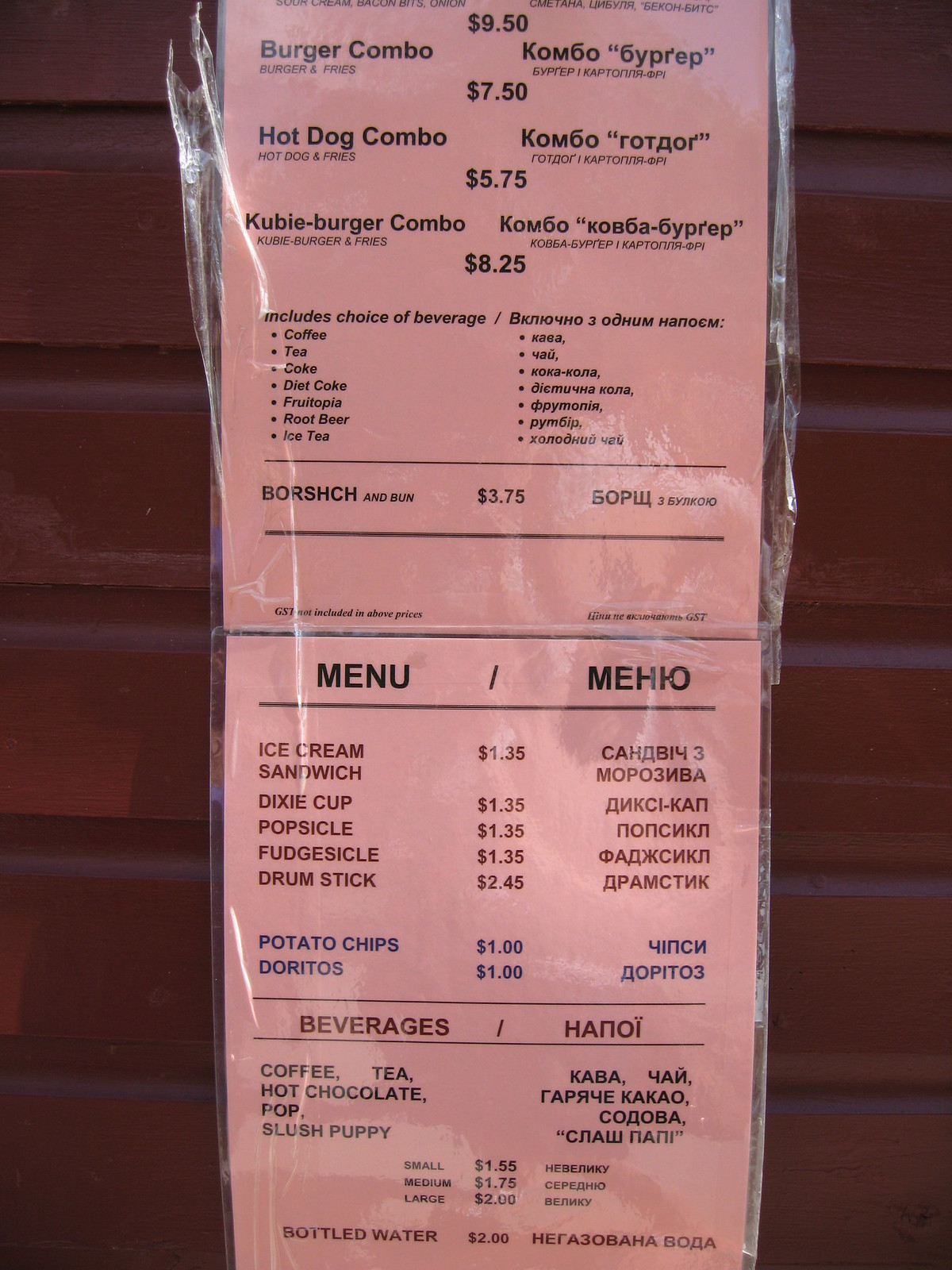This photograph features a menu displaying food and ice cream options. The menu is bilingual, with the left part in English and the right part in another language, possibly Greek or Russian. The offerings include:

- **Combo Meals:**
  - **Burger Combo:** Burger and fries.
  - **Hot Dog Combo:** Hot dog and fries.
  - **Koubi Burger Combo:** Koubi burger and fries.

Each combo includes a choice of beverage: coffee, tea, Coke, Diet Coke, Fruitopia, root beer, or iced tea.

- **Special Items:**
  - **Borscht on a Bun:** Borscht and bun for $3.75.

At the bottom of the menu, additional items are listed:

- **Ice Cream:**
  - Ice cream sandwiches
  - Dixie Cups
  - Popsicles
  - Fudgesicles
  - Drumsticks

- **Snacks:**
  - Potato chips
  - Doritos

- **Drinks:**
  - Coffee
  - Tea
  - Hot chocolate
  - Pop (soda)
  - Slush Puppy

The menu is printed on pink paper and laminated. Most of the text is in black, with some sections, such as the ice cream items, written in red, and the chips and Doritos in blue.